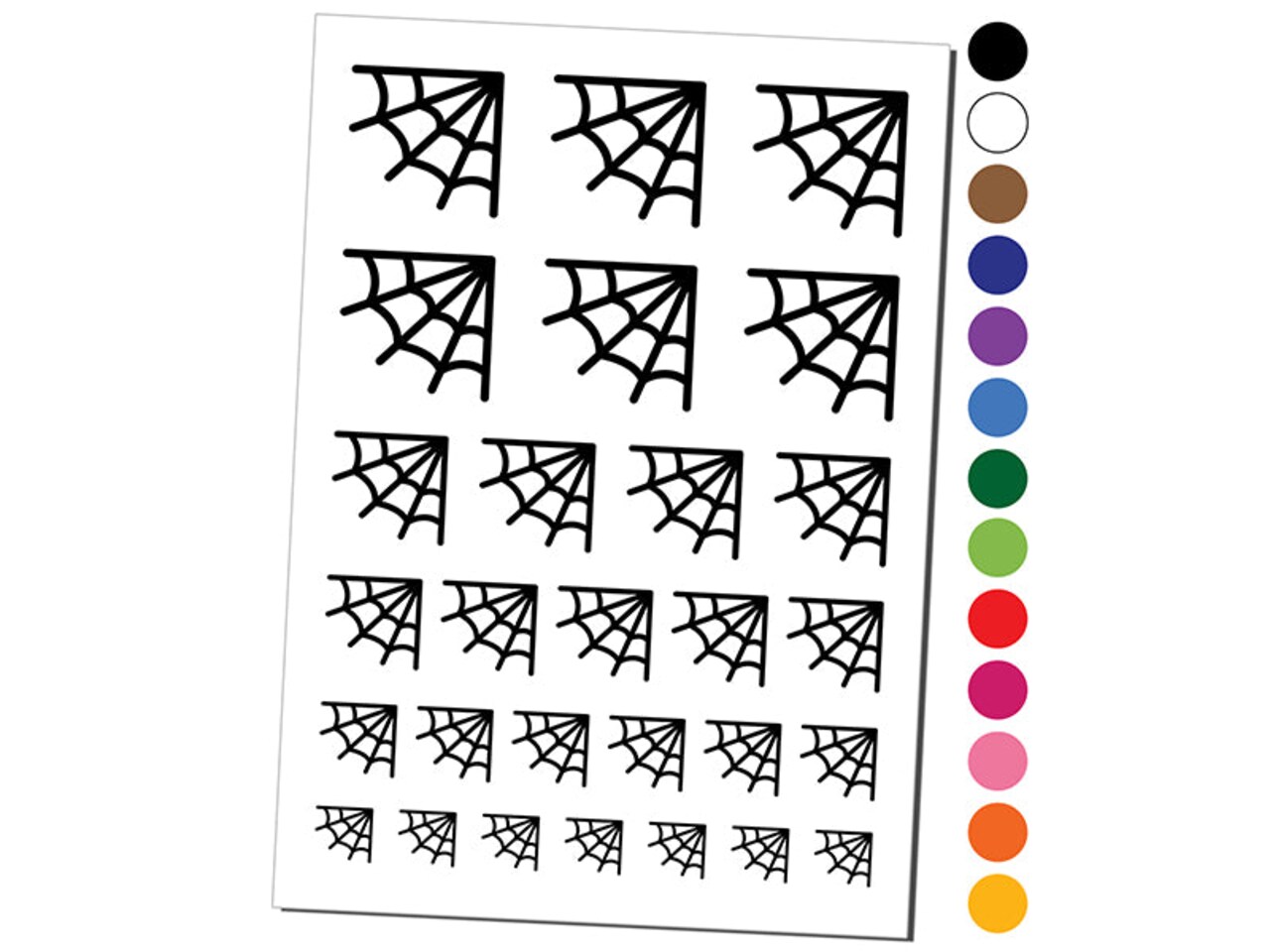This illustrative graphic showcases a white sheet featuring 18 black corner spiderweb drawings arranged by size. At the top, the two largest rows consist of three spiderwebs each, followed by a slightly smaller row of four, continuing with five and six in subsequent rows, and culminating in the smallest representations in a row of seven at the bottom. Each spiderweb emerges from a corner, with straight lines along the top and left edges. To the right of the sheet, a vertical column displays a variety of color options in small circles, starting with black and white, followed by brown, a range of blues and purples, greens, reds to pinks, and ending with orange and yellow. These colors represent potential choices for tinting the spiderweb graphics. Overall, the image presents a detailed visual guide that combines both size variations and possible color customizations for the spiderweb designs.